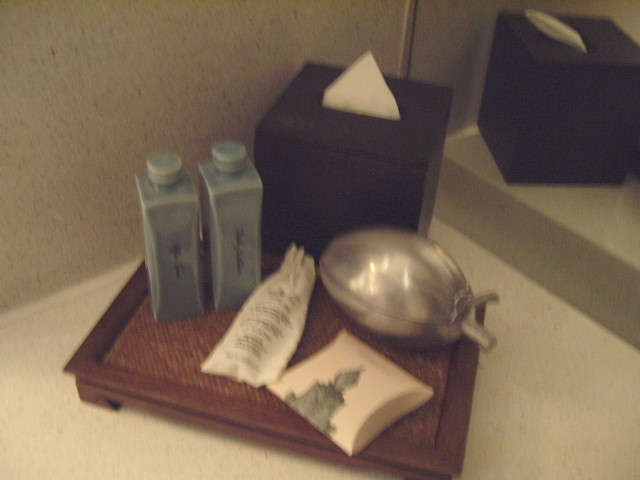A well-organized bathroom countertop features several hygiene products and tools arranged neatly on a wooden tray. The background presents a speckled white and black wall on the top left and a pristine white counter below. A rectangular mirror on the top right reflects the tissue box and other items. The brown, wooden tissue box stands out with a white tissue peeking out from the top. 

Central to the arrangement is a brown, wooden tray holding various items. A prominently placed white piece of paper with a green tree design lies within the tray. A white bag with black writing is situated in the center. To the right corner of the tray, a sleek, stainless steel, egg-shaped item adds a modern touch. Additionally, two twist-off cap bottles, in shades of bluish-green and light gray, complement the scene. 

This detailed setup not only serves practical purposes but also adds an aesthetic charm to the bathroom space.